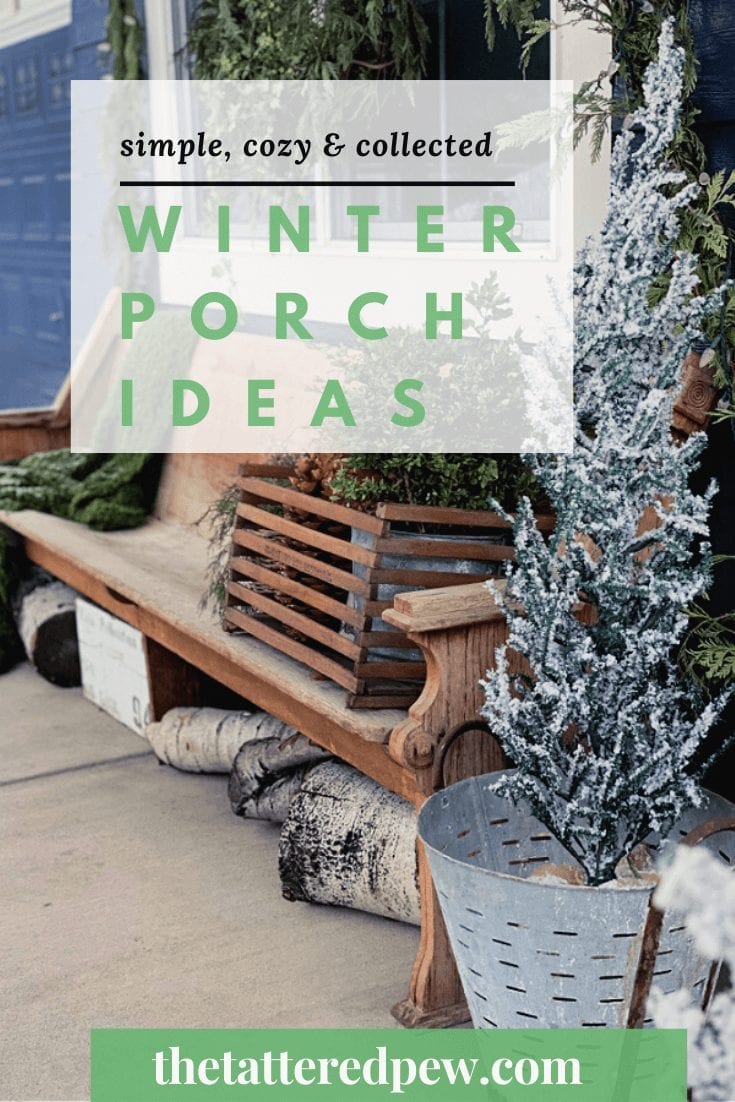This photograph, likely sourced from a website or Pinterest page, features a charming outdoor setting. At the top of the image, black text on a semi-transparent white block reads “simple, cozy, and collected,” followed by green text proclaiming “winter porch ideas.” The bottom of the image centers a green text block that says “thetatteredpew.com.”

The scene showcases a wooden bench with a rustic touch, adorned with a crate and a box filled with plants. Underneath the bench, wooden logs are neatly stacked, enhancing the cozy atmosphere. Beside the bench, a stainless steel bucket holds a small tree that appears to be dusted with snow. The image captures a quaint, winter-ready porch setting, perfect for seasonal inspiration.